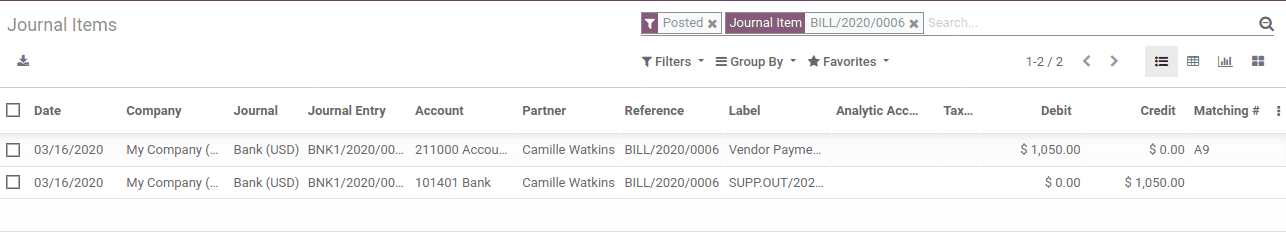The image is a screenshot of a desktop application that heavily resembles a spreadsheet interface. It appears to be a journal management tool. At the top of the screen, there are various menu items including "Journal Items", "Posted Journal Items", and a date range from "2020 to 2020-006". Adjacent to these options is a "Download" button, along with additional tools such as filters and group settings. There is also a section indicating the current page view as "Page 1-2 of 2", accompanied by back and forward navigation buttons.

In the top-right corner, there are buttons likely for changing the format and layout of the view, though their specific functions are not immediately clear. Below this menu, there are two main panel sections formatted similarly to a spreadsheet, organized into several categories: "Date", "Company", "Journal", "Journal Entry", "Account", "Partner", "Reference", "Label", "Analytic Account" (which are both blank), "Tack", "Dot Dot Dot" (both blank), "Debit", "Credit", and "Matching".

In the data entries, the first visible selections have dates of "3-16-2020". These entries seem to be placeholders, as the companies are both generically labeled "My Company". Each row within these selections contains blank cells under several categories, revealing that the fields for analytic account, tack, and additional notes are not filled in.

Overall, the image showcases a structured and detailed view of journal entries within a software tool, providing various functionalities for data management and navigation.